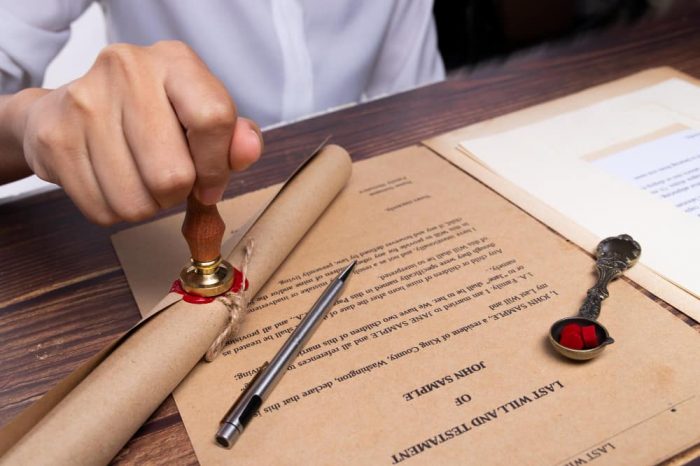This horizontally aligned close-up photograph captures the meticulous act of sealing a document on an older, brown wooden desk with distinctive dark grain patterns. Central to the image is a person's right hand, adorned in a white long-sleeve blouse, pressing a red wax seal onto a rolled piece of brown paper bound with thin twine. The handle of the sealing stamp is brown, clearly showing the red wax being applied. In the foreground, prominently displayed is an upside-down brown document, titled "Last Will and Testament of John Sample," situated alongside a silver pen. The upper right corner reveals additional white papers, providing context to the meticulous and possibly legal scenario depicted. The entire scene exudes a sense of antiquity and careful attention to detail, with the desk's natural wood slats adding a rustic charm.